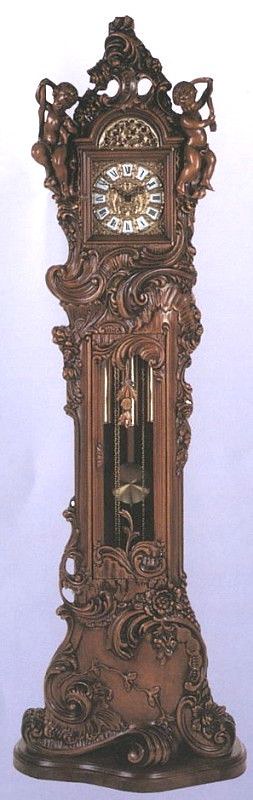This image showcases a highly elaborate and intricately designed grandfather clock, likely an antique piece of significant value. The clock is crafted from dark, richly furnished wood. At the top, there are detailed carvings of small cherubs or putti, appearing to grasp onto branches, giving the impression of a tree motif. The clock face is adorned with ornate golden detailing and features Roman numerals, although the abundance of intricate design elements makes it somewhat difficult to distinguish. The true focus of this masterpiece lies in its ornate body, reflecting exceptional craftsmanship and artistry.